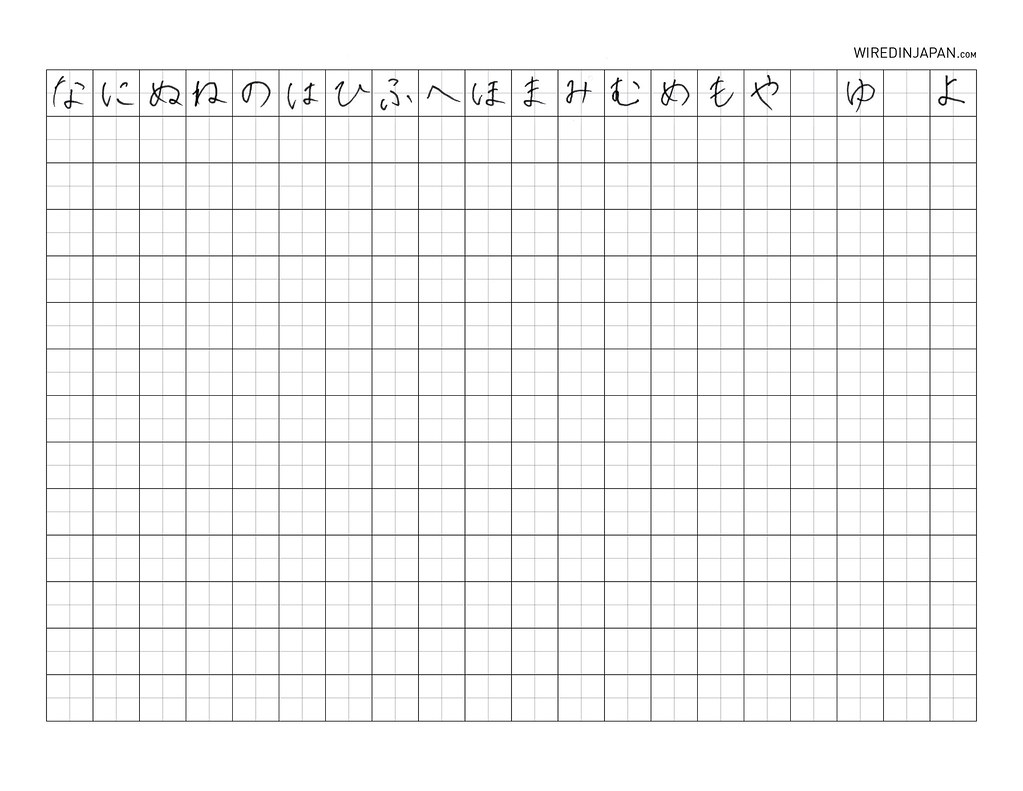The image depicts a piece of gridded paper designed for practicing hiragana writing. The paper features a watermark at the top right, reading "wiredinjapan.com" spelled out in a clear and straightforward manner. The grid is meticulously divided both horizontally and vertically, with each square further subdivided into four smaller squares in lighter-colored ink to aid precision.

This practice sheet specifically focuses on the hiragana syllabary. The first column showcases the character "na," with 13 rows beneath it for learners to practice writing the syllable repeatedly. This pattern continues for the characters "ni," "nu," "ne," and "no."

Following this set, the practice sheet transitions to the next set of syllables: "ha," "ki," "hu," "e," and "ho," each similarly accompanied by 13 rows for writing practice. The layout then proceeds to the syllables "ma," "mi," "mu," "ne," and "mo." 

There are also columns for the syllables "ya," followed by a blank column, "yu," another blank column, and finally "yo." Additionally, it appears that the first row of the grid has some written characters, suggesting that someone has initiated practice but has not yet completed filling out the entire page.